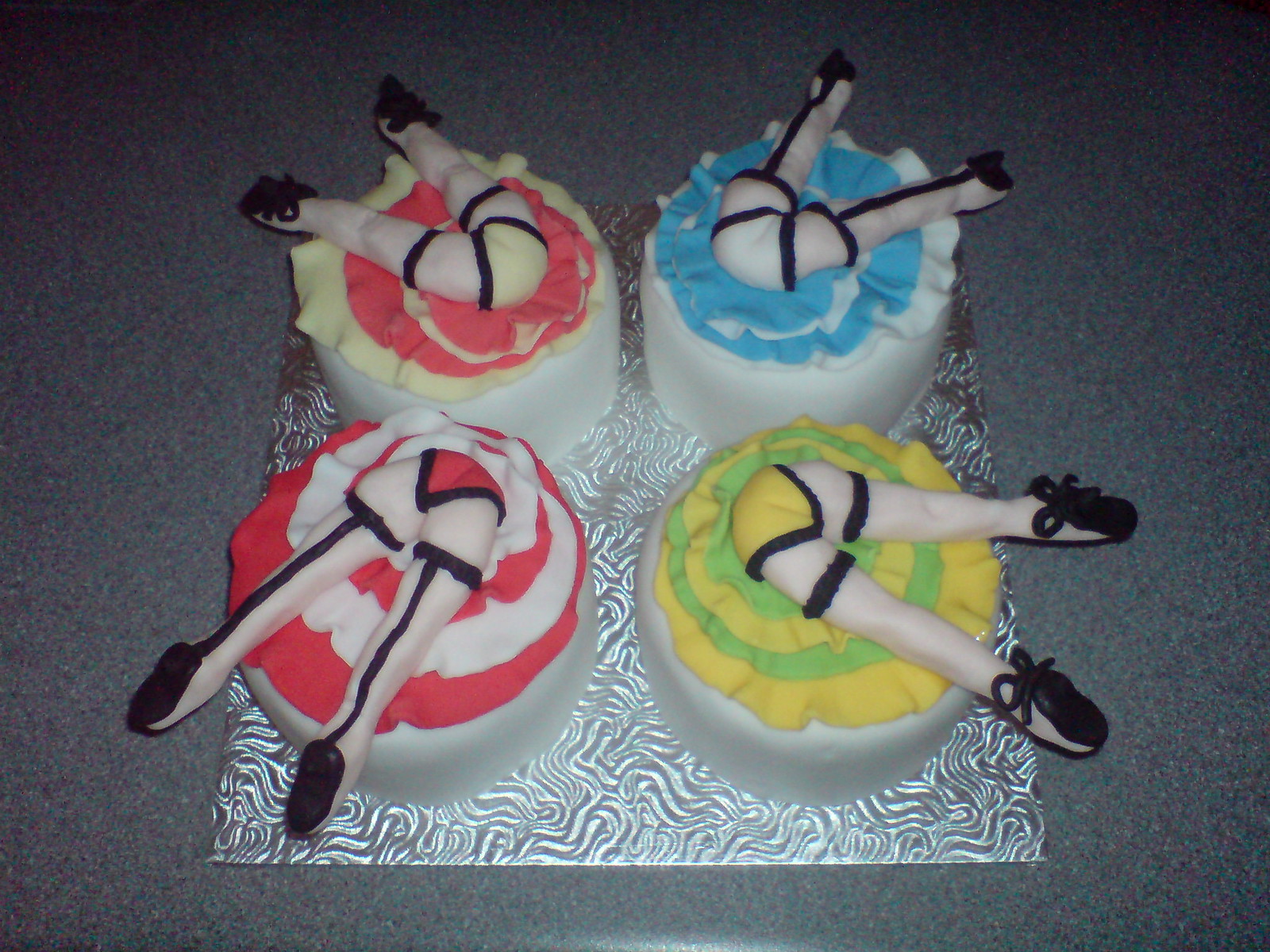This detailed landscape photograph, likely taken indoors on a gray counter or tabletop, features four intricately decorated mini cakes arranged on a square piece of foil in two neat rows of two. Each cake is white with frosted decorations that create the whimsical illusion of a woman having fallen headfirst into the cake, with her legs sticking out in a "V" shape. The decorations depict the woman's exposed bottom, clothed in colored underwear, and her legs adorned with black shoes and stockings. The distinctive skirts, made from frosting, mirror this playful chaos. Starting from the upper left, the cake features a yellow and pink skirt. The upper right cake has a blue and white skirt. The bottom right showcases a skirt with yellow and green hues, and finally, the bottom left has a skirt of red and white. This creative depiction combines humor and artistry, making for a visually striking and amusing image.